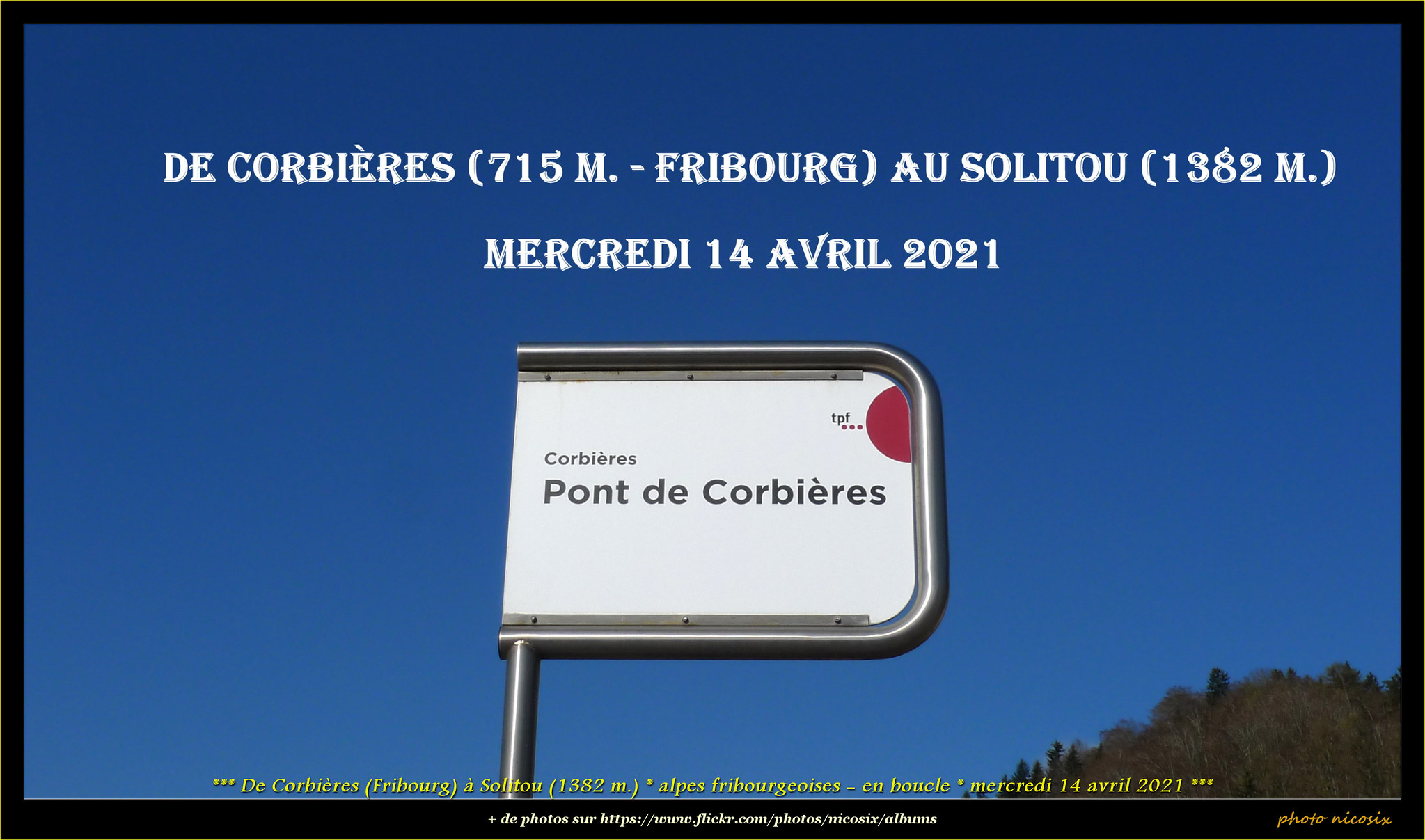This image features an outdoor sign set against a predominantly clear blue sky. The sign, which is white with a silver border and supported by a silver pole, is positioned slightly off-center, giving it a flag-like appearance. In the left-hand corner, you can notice green trees, while the lower right-hand corner also displays some foliage. The sign prominently reads “Corbières Pont de Corbières” in black text, with a distinctive red semicircle in the upper right corner and additional yellow lettering, which is too small to discern. Below this main text, in parentheses, it lists “De Corbière (715 m) – Freiburg en Solitude (1382 m)” followed by “Mercredi 14 Avril 2021,” which translates to Wednesday, April 14, 2021. A website URL, appearing to be from Flickr, and a watermark are present at the very bottom of the image.